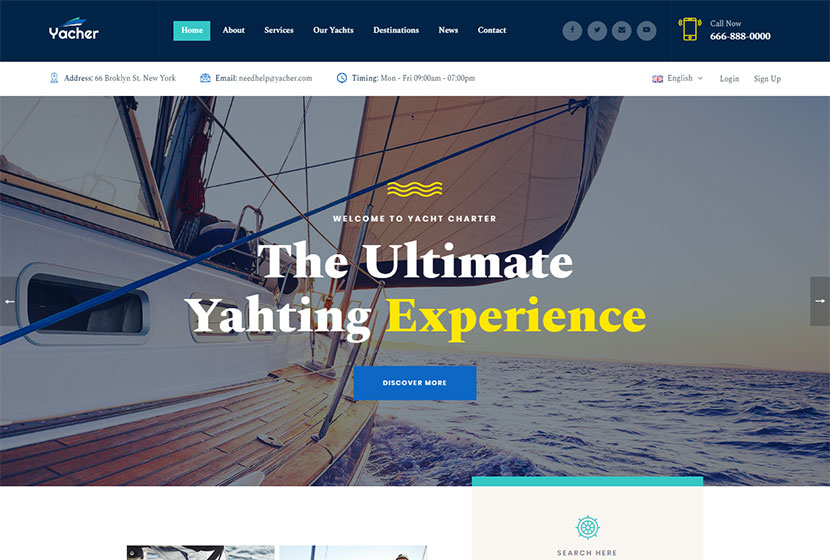The top of the webpage features a dark blue banner, prominently displaying the name "YACHER" in white letters on the left side, accompanied by a small blue logo situated above the text. Centrally located on the page, an image captures a sailboat gliding through the ocean, focusing on its side and the front sail, with a backdrop of expansive, open sea to the right.

Directly beneath the image, bold text welcomes visitors with the phrase “Welcome to Yacht Center,” highlighted by a small yellow wave pattern. 

Further down, a tagline in bold, larger letters states, “The Ultimate Yachting Experience,” with the phrase “the ultimate” in white and “yachting experience” in yellow.

At the bottom of this section, a blue rectangular button with white text invites users to "Discover More," providing a clickable link to explore additional content about the ultimate yachting experience on the YACHER website.